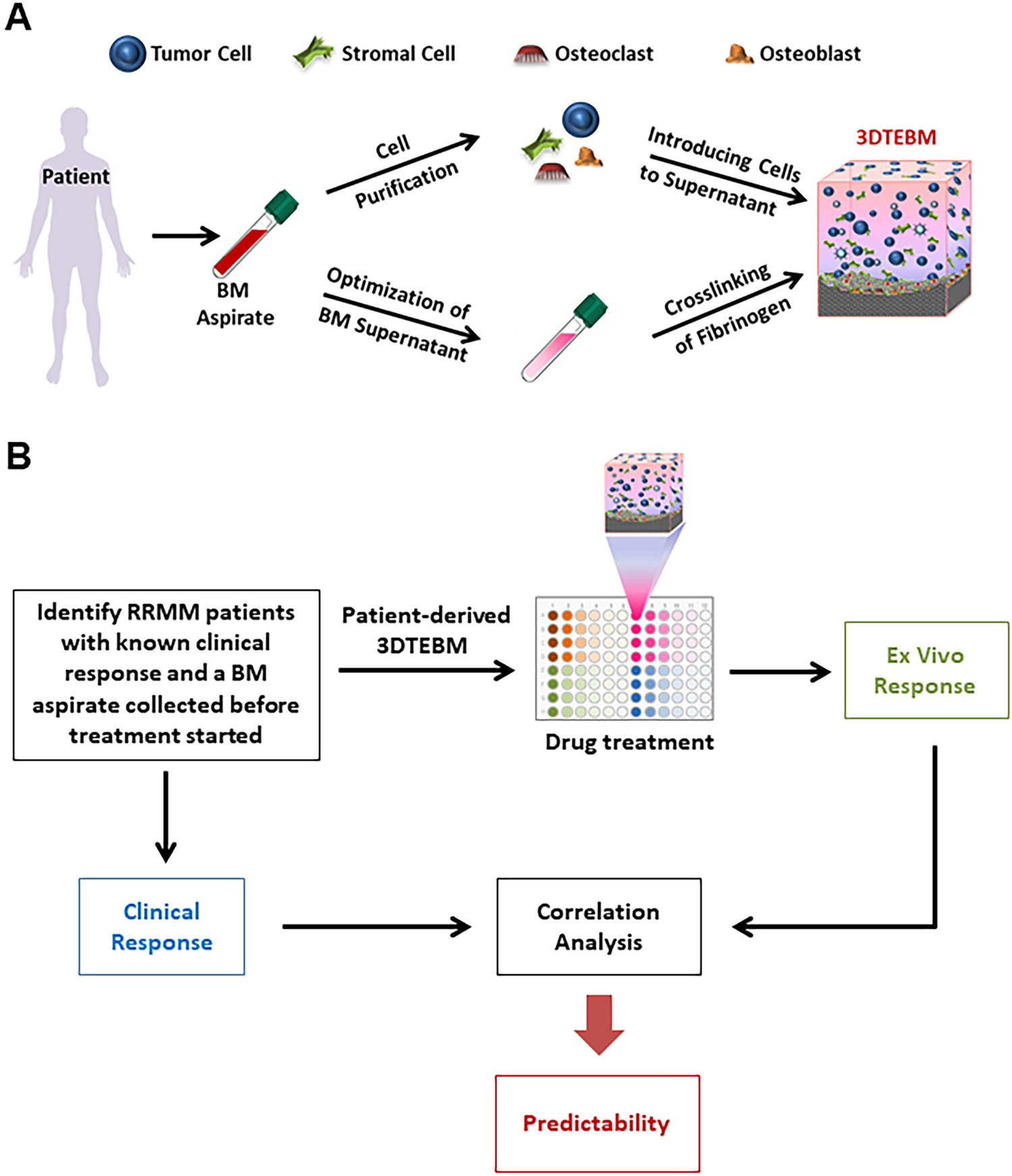The image is a detailed scientific flowchart illustrating the process for handling a patient suffering from a medical condition. It starts at the top with Section A, which depicts an outline of a patient with labels indicating "tumor cell," "stromal cell," "osteoclast," and "osteoblast." An arrow leads from the patient to a BM aspirate (bone marrow aspirate), which then splits into two pathways: one for cell purification and another for the optimization of BM supernatant. The path ends at a block labeled "3DTEBM" (Three-Dimensional Tissue Engineered Bone Marrow).

In Section B, the flowchart begins with a box labeled "Identify RRMM patients with known clinical response and a BM aspirate collected before treatment started." This box points to another labeled "clinical response" and a separate box for "correlation analysis." A right-pointing arrow directs to "ex vivo response," leading to a final arrow connected to "predictability." Additionally, a large box with numerous colored dots representing cell dyes is featured within this section, highlighting the complex nature of the analysis.

Throughout the flowchart, there are various diagrams of cells and test tubes to visually represent the different stages of the process. The key steps include the identification of the patients, collection and preparation of the BM aspirate, cell purification, optimization, drug treatment, and the subsequent analysis to predict clinical responses.